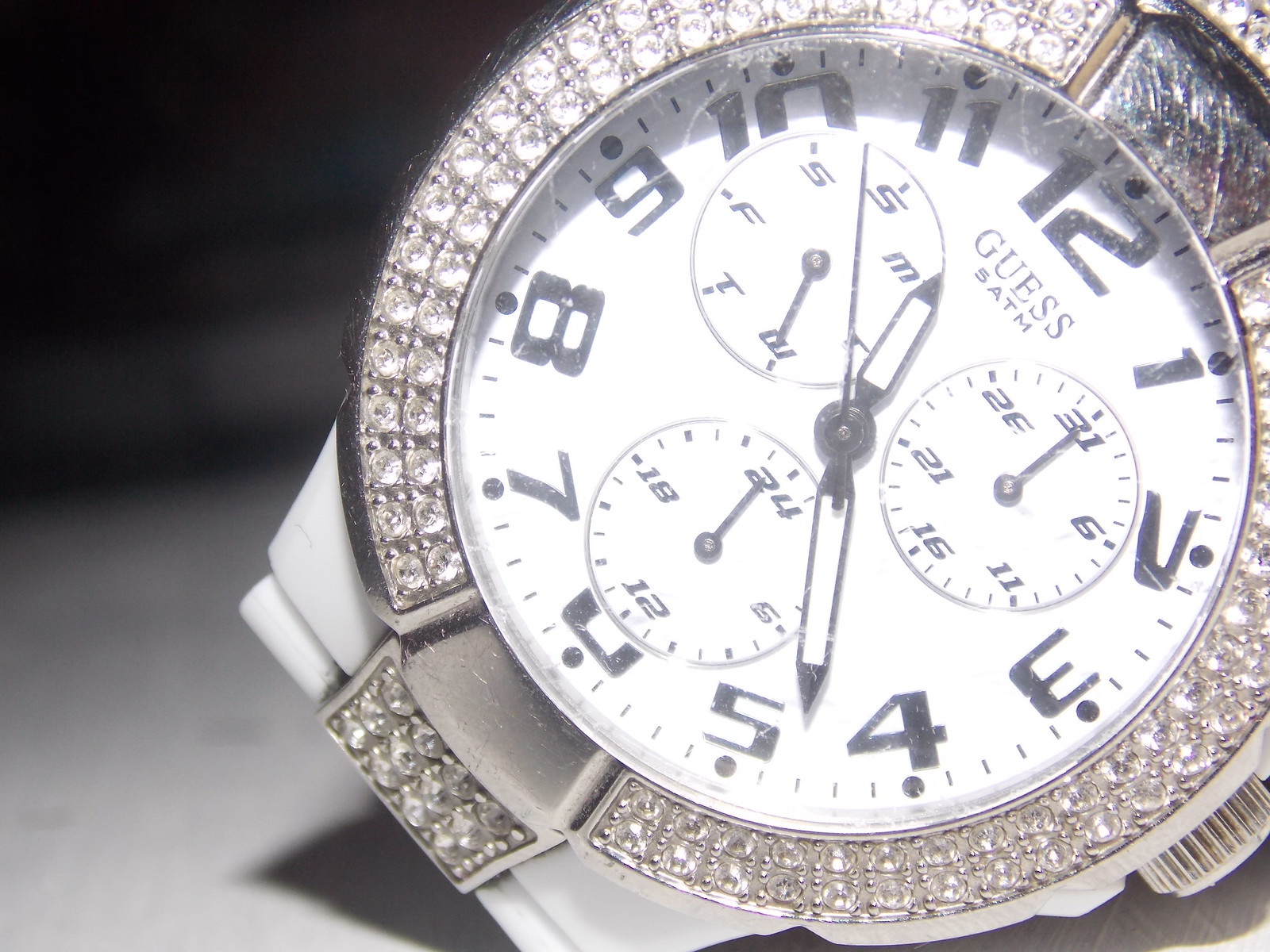A close-up image of a luxury wristwatch from Guess. The watch features a pristine white dial framed by a clear case that offers a glimpse of its intricate design. Encrusted with two rows of sparkling diamonds along the bezel, the timepiece exudes elegance and sophistication. The dial displays standard Arabic numerals rather than bolded ones, ensuring legibility and classic appeal. Additionally, the watch face includes three subdials, designed as miniature clocks, providing functionality and a complex aesthetic. The main hour and minute hands are prominently displayed, indicating the time is precisely 11:19.